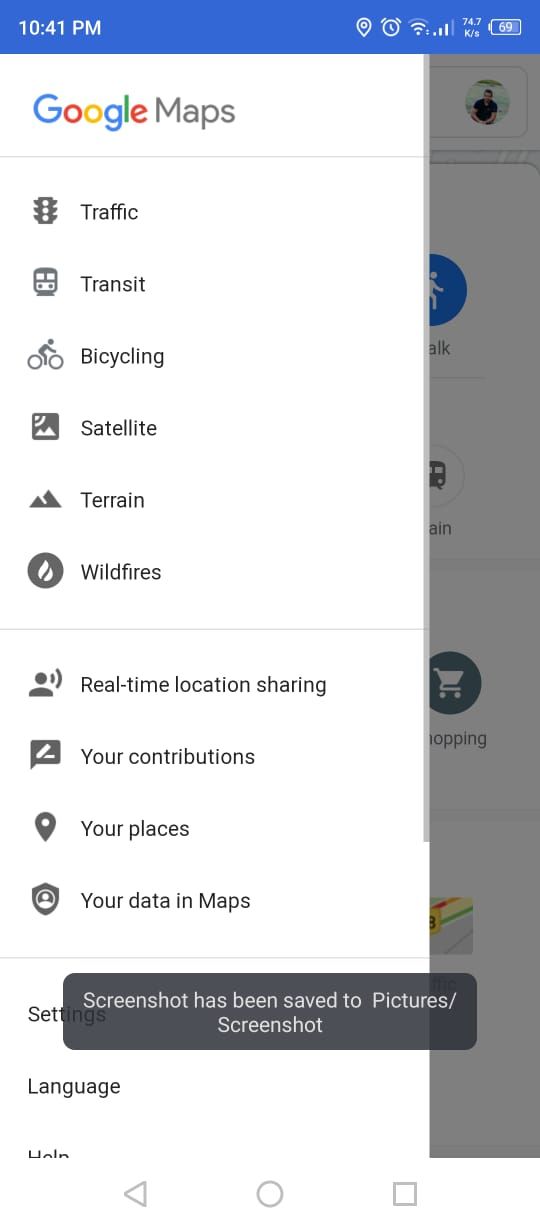The image is a screenshot captured from a mobile device, displaying the Google Maps application interface. At the top of the screenshot, there's a blue status bar where the left side shows the time as 10:41 PM. On the right side of this bar, several icons are aligned from left to right: the location icon, the alarm icon, the Wi-Fi icon, the network icon, and the battery icon indicating 69% charge.

Beneath the blue status bar, the Google Maps logo is visible, with the word "Maps" next to it. Below the logo, a set of options is presented, neatly arranged in a vertical column. These options are:

1. Traffic
2. Transit
3. Bicycling
4. Satellite
5. Terrain
6. Wildfires
7. Real-time location sharing
8. Your contributions
9. Your places
10. Your data in Maps

Each option is written in dark grey text, making it easily readable against the background.